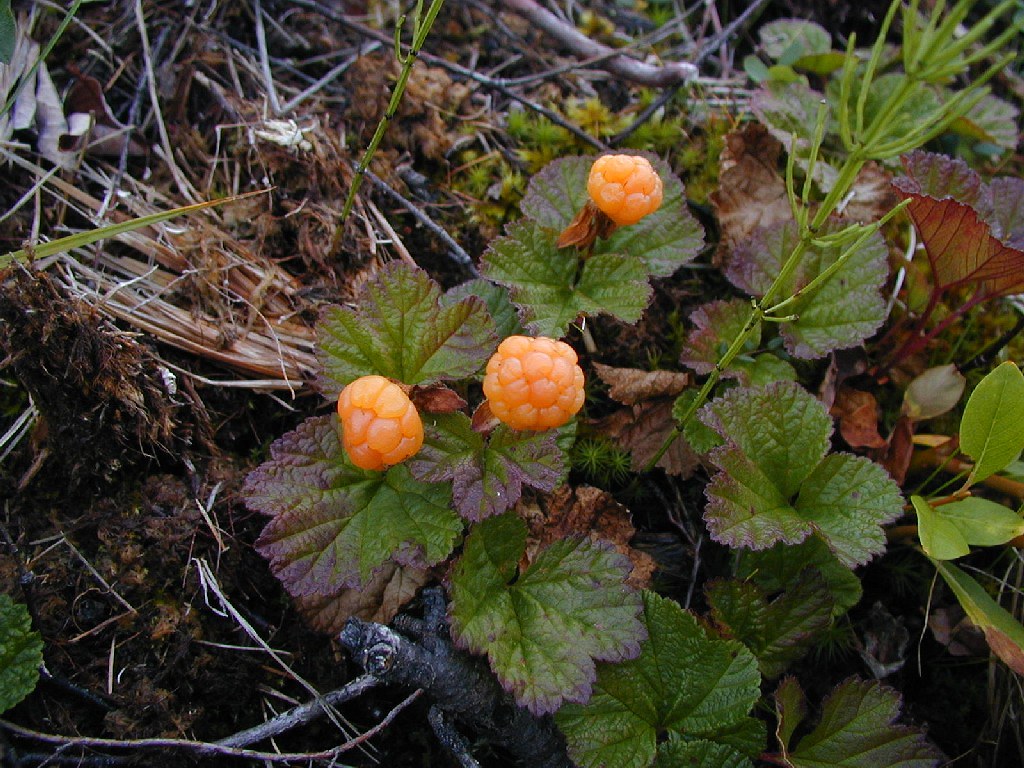The photograph captures a detailed view of a forest floor teeming with natural elements. At the center and slightly to the left, there are several clusters of orangish, raspberry-shaped berries, each comprised of tiny bulbs. One berry is prominently in the center, another just left of center, with a third above and slightly to the right of it. The berries are surrounded by green leaves, which transition to darker hues at the edges and feature purple tips. Below and to the right of the berries are additional green leaves, sticks, and brush. A piece of weed extends upward and to the right, adding to the intricate forest floor tapestry. The ground appears wet, suggesting recent rain, with visible dirt, twigs, and fallen branches scattered throughout the scene, especially noticeable in the bottom left-hand corner.